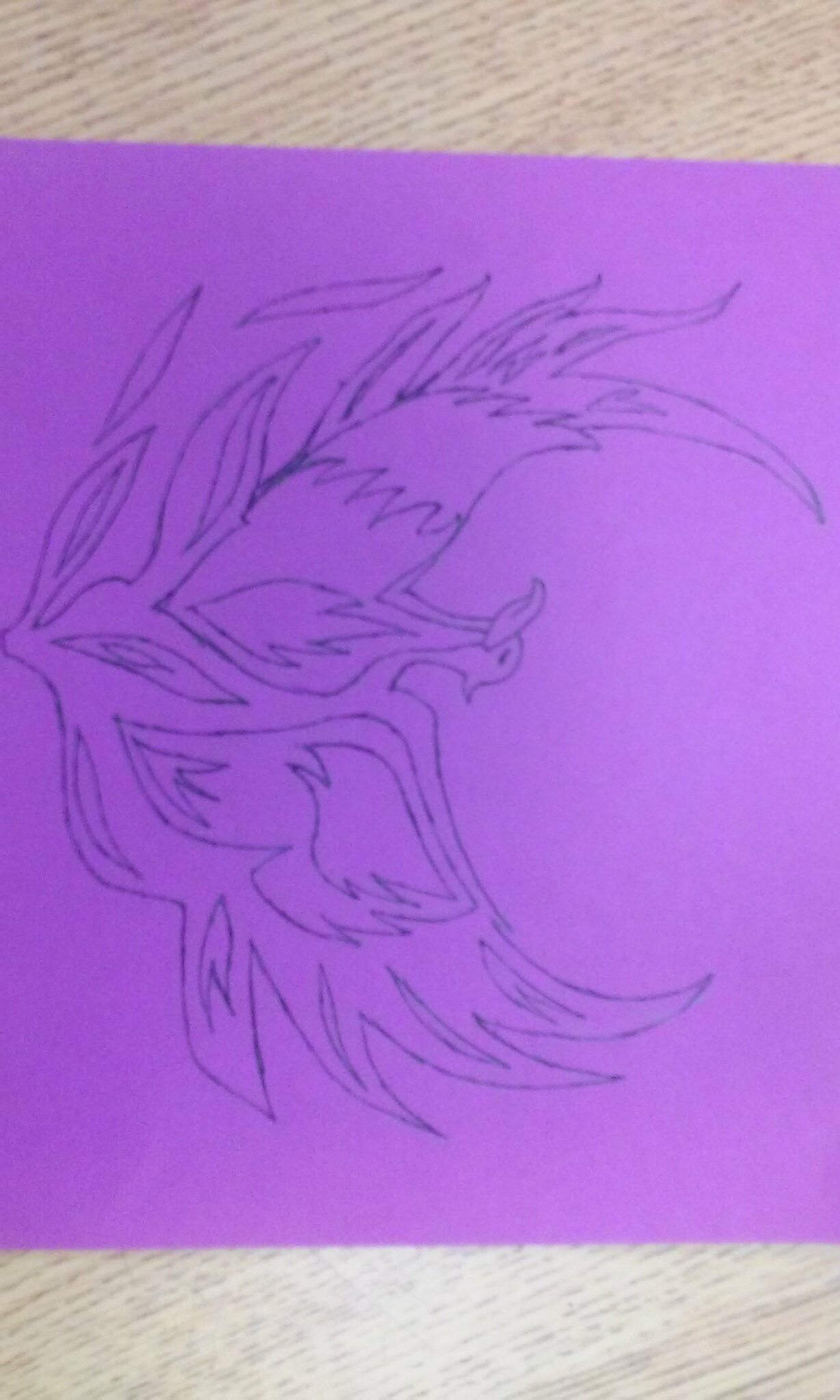This image features a detailed drawing of a bird-like creature, rendered in black ink on a purple sheet of paper. The drawing is oriented sideways in the photograph. The bird has a prominent beak and simple line representations for its eyes. Both wings are depicted as spread out, showcasing intricate feather details. The purple paper rests on a tan platform with a wood grain pattern. The composition focuses solely on the creature and its surroundings, highlighting the artistry and choice of materials used in the drawing.